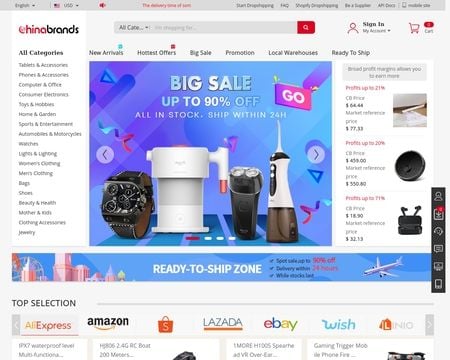Here is a detailed and cleaned-up caption for the described image:

"In the photograph, we see a vibrant screenshot of a colorful web page featuring a variety of hues, including white, purple, blue, pink, and black. The page prominently displays the word 'China' in red text and the phrase 'it's brands' in black underneath. The currency is set to US dollars. The header section includes options for 'Start,' 'Fax,' and 'All Documents,' as well as a sign-in option represented by a red account user icon. The shopping cart icon indicates that it is currently empty. 

On the left side of the page, a menu lists categories such as tablets, phones, computers, hobbies, sports, lighting, women's clothing, men's clothing, and bags. Featured products are showcased in the center of the page against a colorful background of blue, purple, and pink shades, with a bold banner announcing 'Big Sale up to 90% off.' This is accompanied by the phrases 'All in stock' and 'Ship within 24 hours,' along with a call-to-action button labeled 'GO' in a pink rectangle. 

Highlighted products include a flosser, an electric shaver, a watch, and what appears to be an ice cream maker. At the bottom of the screen, banners for popular e-commerce platforms Amazon, Lazada, eBay, and Wish are visible."